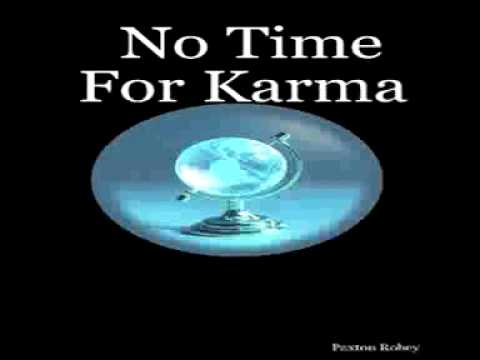The image is a book or album cover set against a solid black background, suggesting an outer space theme. Centered at the top is the title in white, Times New Roman font, "No Time for Karma", with "No Time" on the top row and "For Karma" on the row below. Directly below the title, there's a blue, slightly flattened oval enclosing a light blue globe, similar to a desk globe on a stand, appearing slightly distorted. The globe is mounted on a metal base. In the bottom right corner, there's a blurred signature of the artist whose name seems to read as Preston R. or something similar.